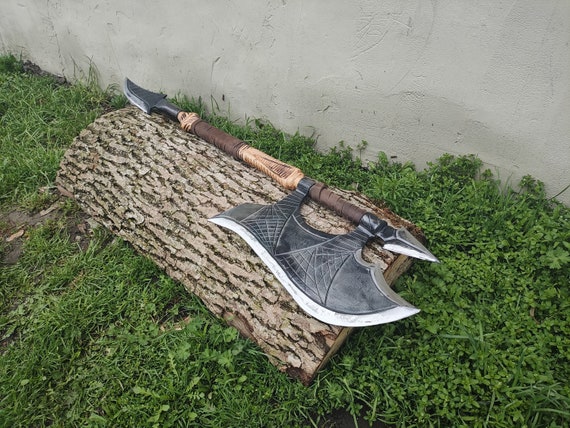In this photograph, we are presented with a detailed scene featuring a medieval-style axe displayed in a natural, unmanicured outdoor setting. The ground is covered with weedy grass, and leaning against a gray cement wall lies a large, aged tree trunk, showcasing its intricate bark and grain details. Nestled on this half log is the focal point: a formidable and ornate fighting axe, likely a collectible. This antique weapon features a gray metal head with detailed engravings, its sharp edges gleaming silver. Both ends of the handle are adorned with dagger-like points, one at the top and another curved one at the bottom, also made of metal. The handle itself is crafted from engraved wood, displaying a mix of dark brown and light tan hues. This axe undeniably evokes a sense of historical weaponry, designed for serious combat rather than simple woodworking.